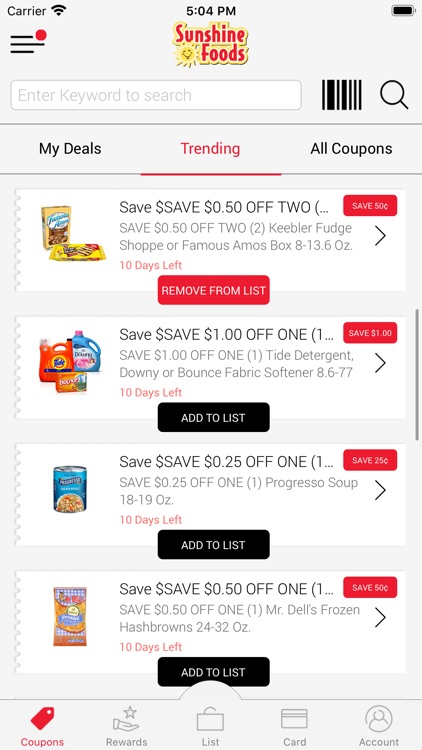**Detailed Caption:**

This image is a screenshot from a mobile device displaying the Sunshine Foods app, which offers various coupons. 

At the top of the screen, typical status icons are visible: the word "Carrier" on the left, a Wi-Fi connected symbol next to it, the time displayed in the center as 5:04 PM, and a horizontal battery icon on the top right, all in black. The background for the phone screen and the app itself is light gray.

Directly below this is a row containing a hamburger menu icon (three horizontal lines) on the far left, with a red or pinkish notification circle indicating an alert. In the center is the Sunshine Foods logo, which features a pink emblem with a yellow sun outline. To the right of this, there's a search bar with the placeholder text "Enter a keyword to search," enclosed in a thin gray border. Adjacent to the search bar are barcode and search icons.

Beneath this row is a thin black line, followed by a tab menu which includes "My Deals," "Trending," and "All Coupons." The "Trending" tab is highlighted in pink and underlined, indicating it's the active tab.

The main content of the screen displays four rows of products, each set on a white rectangular background with a perforated left edge, all set against the gray background of the app. 

1. The first row features a product image of Famous Amos cookies. The text reads "Save $0.50 off 2…" with a pink button saying "Save 50 cents" in white text. Further details indicate "Save 50 cents off 2 Keebler, Fudge Shoppe or Famous Amos boxes (8-13.6 ounces). 10 days left. Remove from list." A greater-than symbol hints at additional options.

2. The second row offers a coupon for Tide detergent, Downy, or Bounce fabric softener, stating "Save $1 off 1" with a similar pink button labeled "Save $1." Details say "Save $1 off 1 Tide detergent, Downy, or Bounce fabric softener (8.6 to 77 oz). 10 days left. Add to list."

3. The third row features Progresso soup under the same format.

4. The fourth row highlights Mr. Dell's frozen hash browns.

At the bottom of each product row is a black button with "Add to list" in white letters, and similar options to add or remove items from the list.

The app's main navigation menu is located at the bottom of the screen, from left to right: "Coupons" with a tag icon, "Rewards" with a hand holding a star, "List" with a suitcase/padlock icon in the center, "Card" with a credit card icon, and "Account" with a circle and person outline icon.